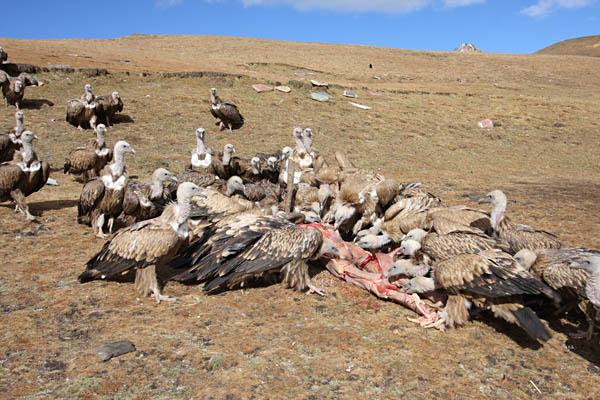This outdoor scene captures a stark, barren landscape looking upward from the base of a hill. The land is scrubby with patches of light tan, dead grass, and there is a thin slice of a clear, blue sky adorned with just hints of white clouds at the very top of the frame. Dominating the image is a large group of turkey vultures, approximately 30 to 40 in number, either feeding on or approaching a carcass, the specifics of which are unidentifiable but gruesomely exposed with red bloodied flesh and innards visible. The turkey vultures, characterized by their white heads, off-white beaks, black eyes, and sharp talons, have thick, muscular legs and wings that display a mix of white and light beige feathers, while their short tail feathers range in color from black to dark gray. All of the birds are grounded, some actively pecking at the carcass with their white feet, others making their way toward the feast, contributing to the unsettling yet compelling nature of this wilderness scene.